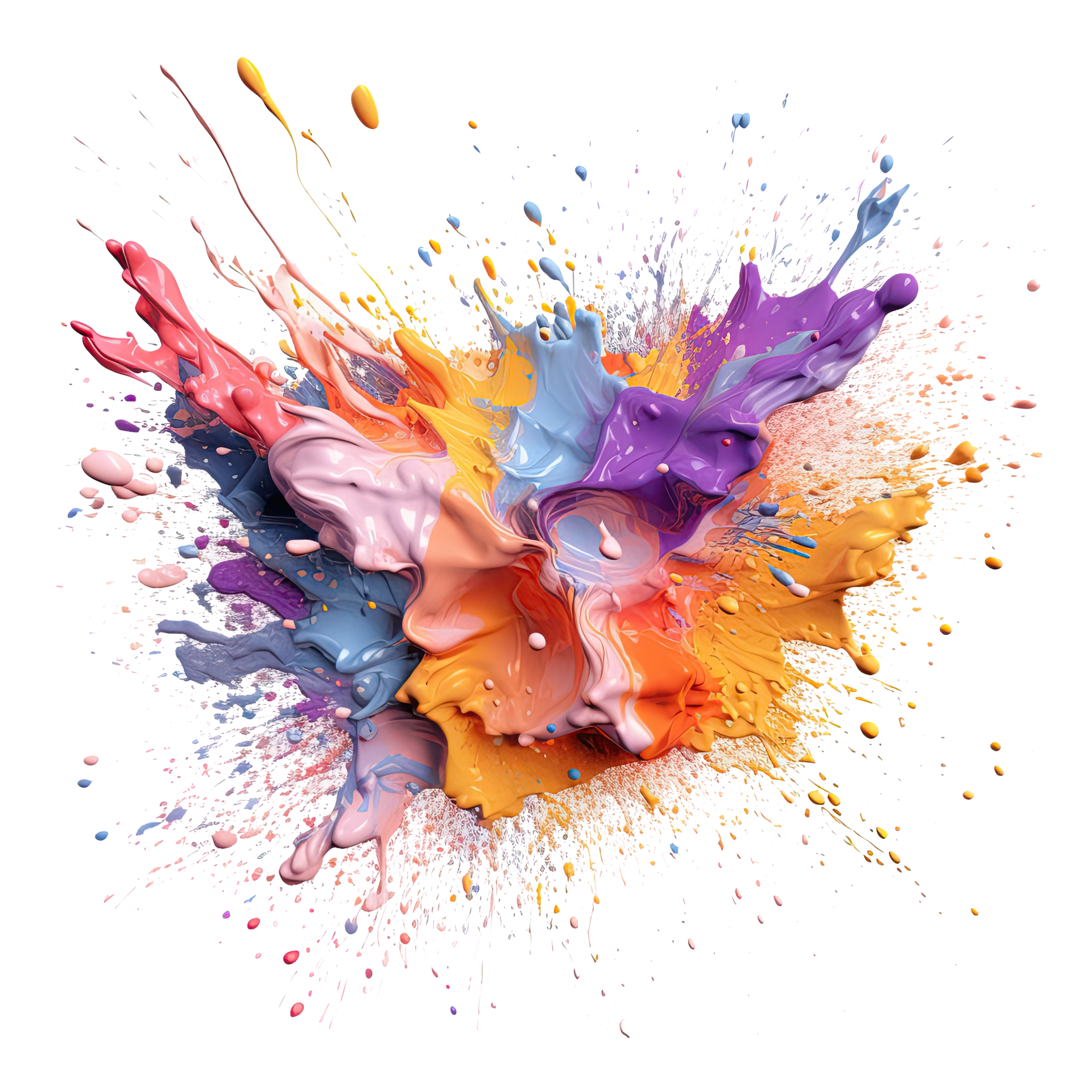The image captures the dynamic and vibrant moment of a paint splash on a stark white background, creating a striking, abstract visual. Thick, multicolored paints, likely acrylic or latex, radiate from a central impact point, forming a dramatic explosion of hues. Dominant colors include purple, light blue, orange, dark yellow, shades of pink, and a peachy pink, interspersed with a unique mauve tone. The paint appears to have been forcefully thrown, with droplets of varying sizes—ranging from tiny specks to elongated strands—flying outward. The photograph gives a strong three-dimensional impression, emphasizing the suspended motion as if captured in mid-air. The composition evokes the energetic and chaotic style reminiscent of Jackson Pollock’s splatter paintings, with the paints mingling and splashing in every direction, creating an immersive and kinetic scene.